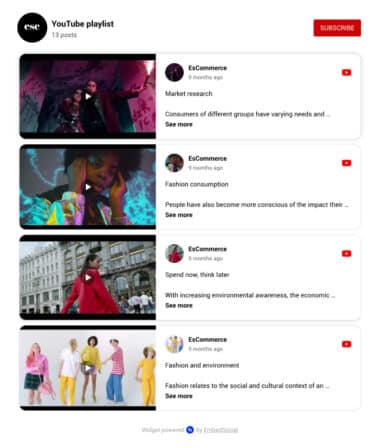The screenshot displays a YouTube playlist interface against a white background. The interface is organized into four distinct rows, each featuring a thumbnail image on the left and corresponding playlist details to the right. Additionally, a prominent red "Subscribe" button is located in the upper right corner of the display. On the upper left side, a black circle is visible, accompanied by the text "YouTube Playlist" written in black.

The thumbnail images portray various individuals engaged in different activities. The fourth image in the bottom row notably depicts a group of five people. Starting from the left, the lineup includes a woman dressed in a pink sweater and blue tartan skirt. Beside her stands a man wearing yellow pants and a white shirt. Next in line is a woman clad in a light brown mini dress, and finally, a woman in a pink top paired with blue pants completes the group.

Overall, the varied attire and activities depicted in the thumbnail images suggest that the playlists encompass a wide array of content, appealing to diverse interests and preferences.